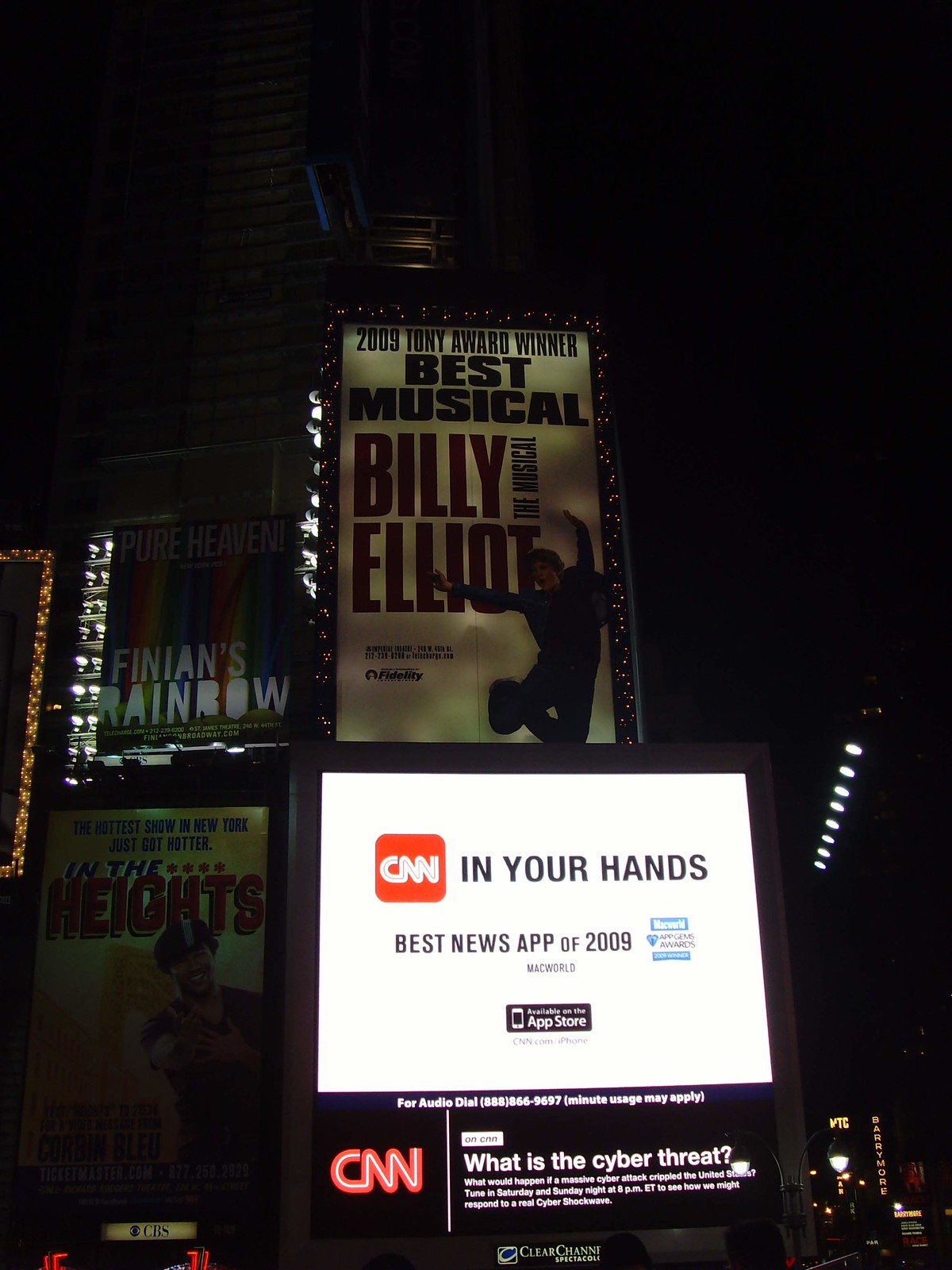The image captures the vibrant nightlife of a theater district, likely resembling a place like Times Square. Dominating the scene are several illuminated posters and display screens promoting theater productions and advertisements. At the center foreground, a brightly lit screen advertises CNN's "Best News App of 2009," highlighting a headline that reads, "What is the cyber threat?" flanked by the CNN logo. Behind this screen, a large, brilliantly lit poster for the musical "Billy Elliot" stands out, showcasing the 2009 Tony Award winner for Best Musical with a boy joyfully leaping in the air, surrounded by an array of lights. To the left of this is the colorful poster for "Finian's Rainbow," set against a rainbow background and captioned "Pure heaven." Further left is another theater poster for "In the Heights," featuring an image of a person looking at the camera. The scene is framed by the glow of city lights, including those from a nearby building visible in the background, enhancing the lively atmosphere of this bustling theater district at night.